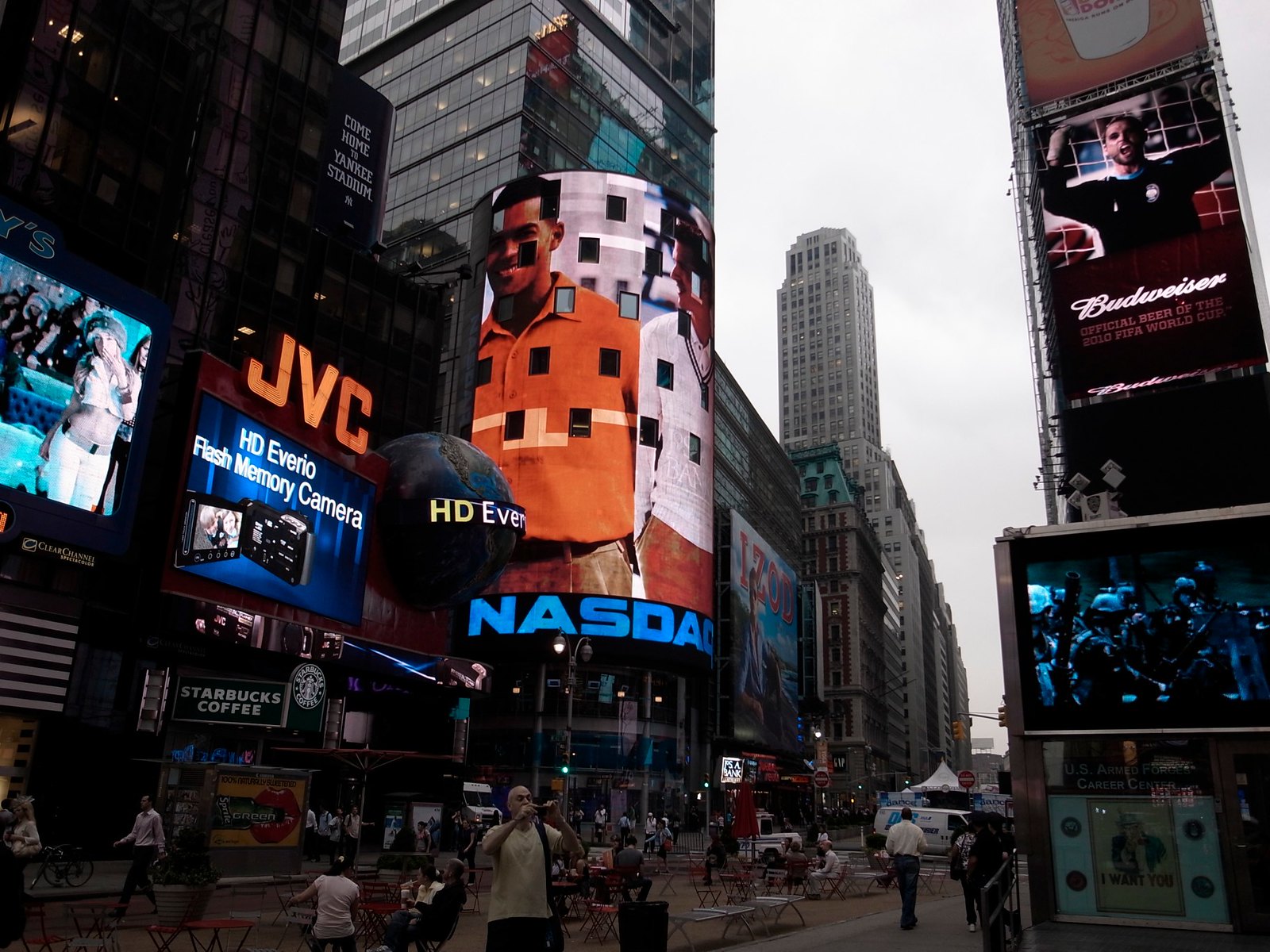The image captures a bustling street in Times Square, New York City, lined with towering skyscrapers that cast a shadow over the scene below. Central to the composition is a large NASDAQ banner featuring a man in an orange shirt with black hair adjacent to a person in a white shirt, both adorned with black squares. Above the NASDAQ sign, grey windows climb to the top of the skyscraper, which is crowned with a lighted chandelier. The sky is overcast, hinting at a cool, possibly autumn day.

To the left of the NASDAQ ad, a lit-up JVC billboard promoting a "HD Vario flash memory camera" stands prominently, accompanied by a globe graphic. Adjacent, a partial TV screen shows a woman in white attire, a heavy scarf on her head, with a large bare midriff. On the far right, an orange advertisement for JVC is followed by a Budweiser sign, adorned with cursive writing and the image of a man in a black shirt with his mouth open, hands raised. Below, in the midst of the lively street, a man in a yellow shirt is seen capturing the moment with his camera, embodying the tourist spirit in this iconic cityscape.